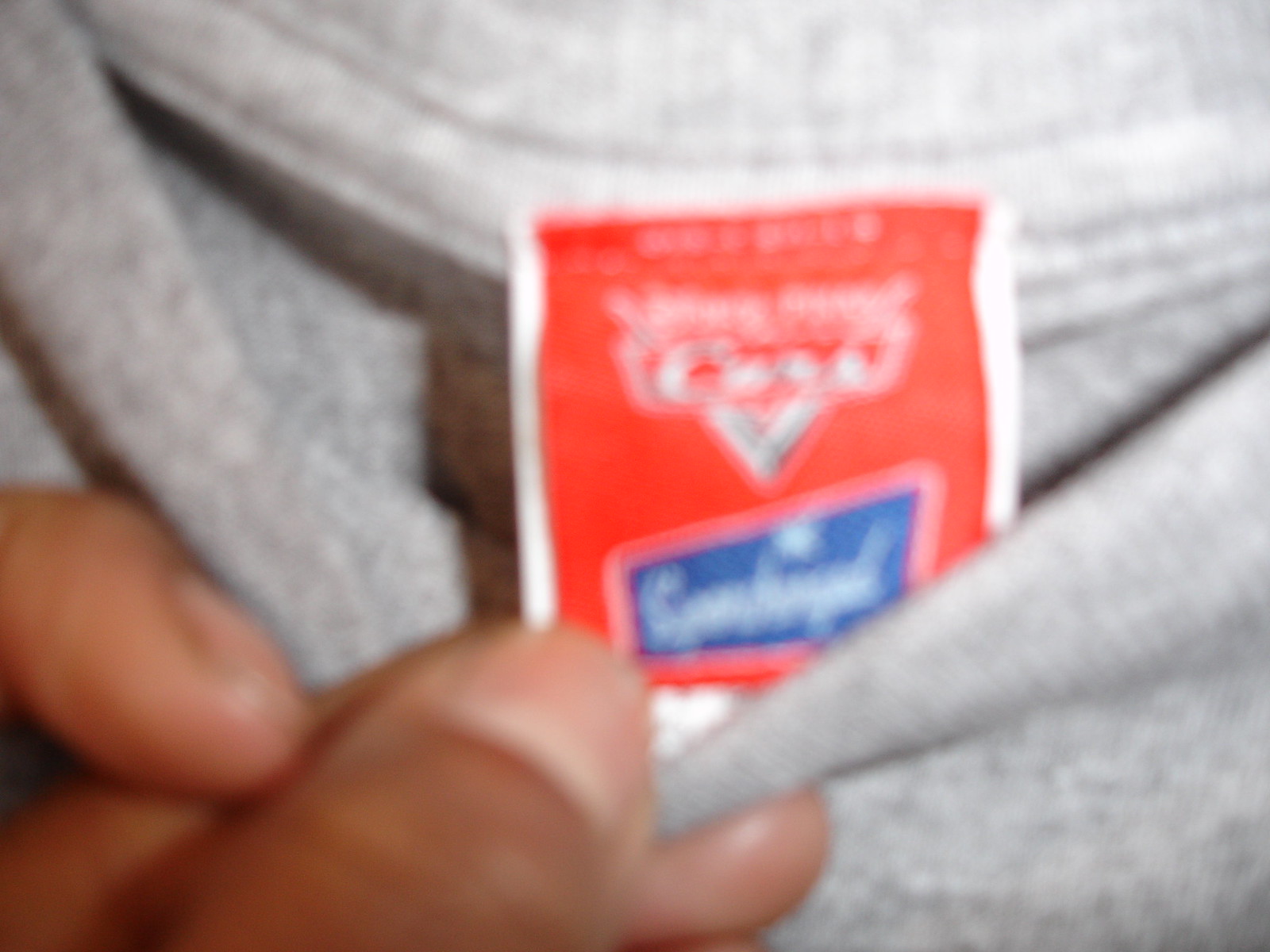This image, although blurry, depicts a piece of heather gray clothing, possibly a shirt. In the lower left corner, a hand is visible, holding a red tag. The tag features white trim along three edges, with the top edge left untrimmed. Despite the blurriness, the tag shows a brand name in blue with a white font, accompanied by a white logo above it. The hand is gripping the tag with the thumb placed on top and one finger beneath the fabric, while another finger can be seen to the left, aiding in holding the garment steady.